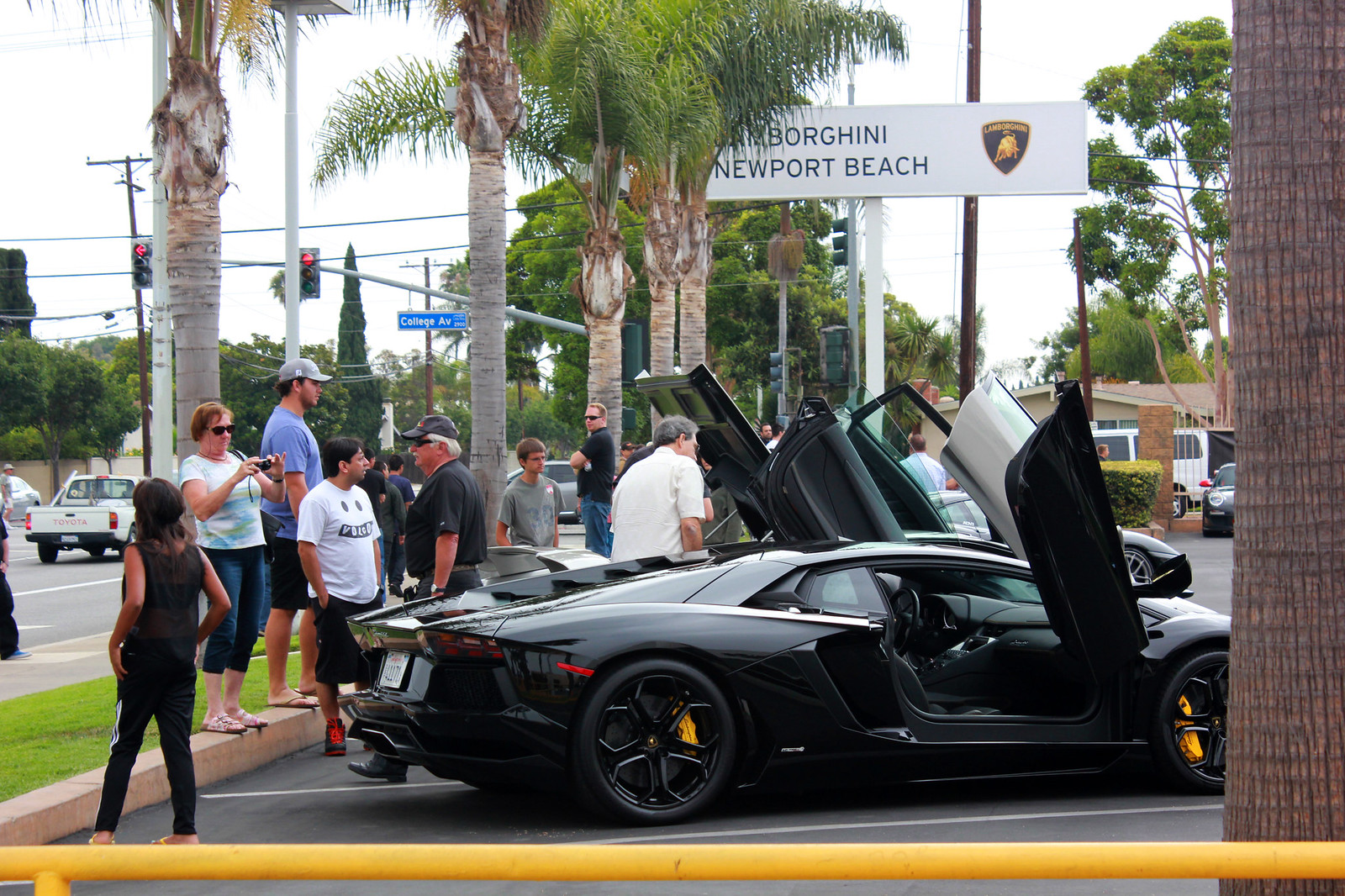The image captures an outdoor setting at a Lamborghini dealership in Newport Beach, California, where several luxury cars are on display in a parking lot. Dominating the foreground is a sleek black Lamborghini with its iconic scissor doors flung open upwards towards the sky. Beside it, more Lamborghinis in various colors, including silver, also have their doors open. A white sign above the scene reads "Lamborghini Newport Beach." It's a sunny daytime scene, illuminated by the bright sky. Palm trees line the background, accompanied by a grassy area and a street busy with traffic and traffic lights. In the parking lot, at least ten people stand around, some peering inside the cars and others taking photos, while a man is notably inspecting the interior of one vehicle. The engaging environment is typical of sunny Newport Beach, providing a luxurious yet relaxed atmosphere.